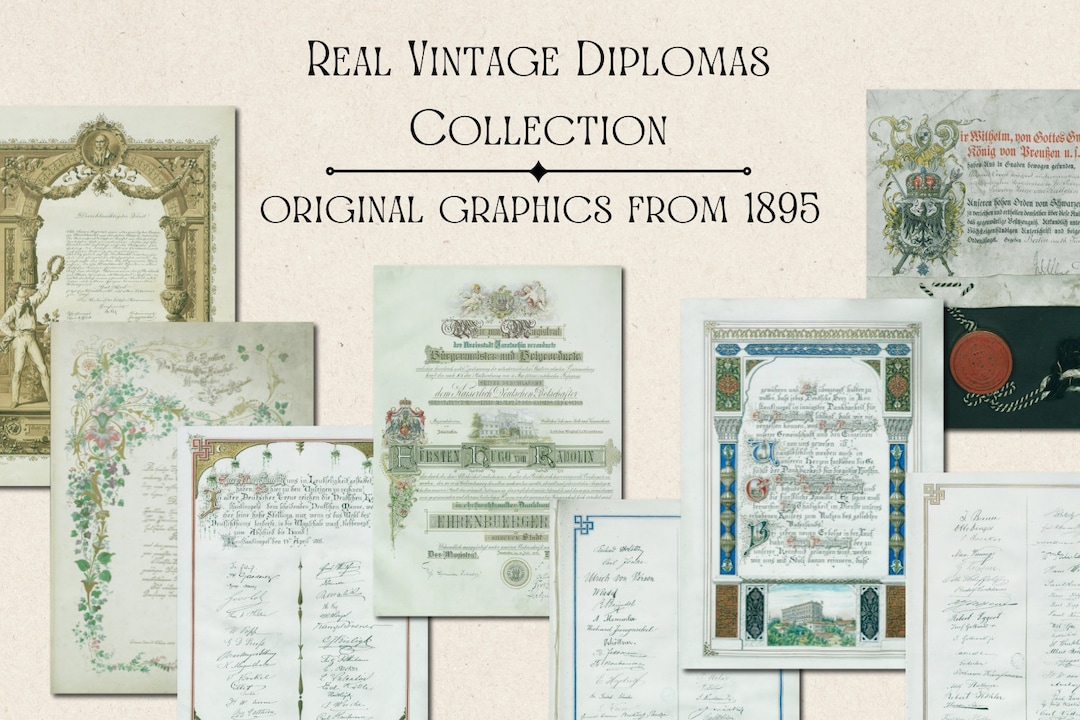This advertisement showcases a "Real Vintage Diplomas Collection" featuring original graphics from 1895. The image's centerpiece is a description in an antique font, framed against a background reminiscent of old building paint. Eight vintage diplomas, stacked haphazardly, surround this description. The diplomas are highly ornate, each adorned with intricate illustrations alongside elaborate text. Notable examples include a diploma on the left with an intricate gold design and a cowboy holding a lasso in the bottom left corner, another beneath it encircled by flowers and vines, and a top right diploma in a Victorian font accompanied by a crest. The diplomas, while too small in resolution for their text to be legible, visually convey a rich historical aesthetic.